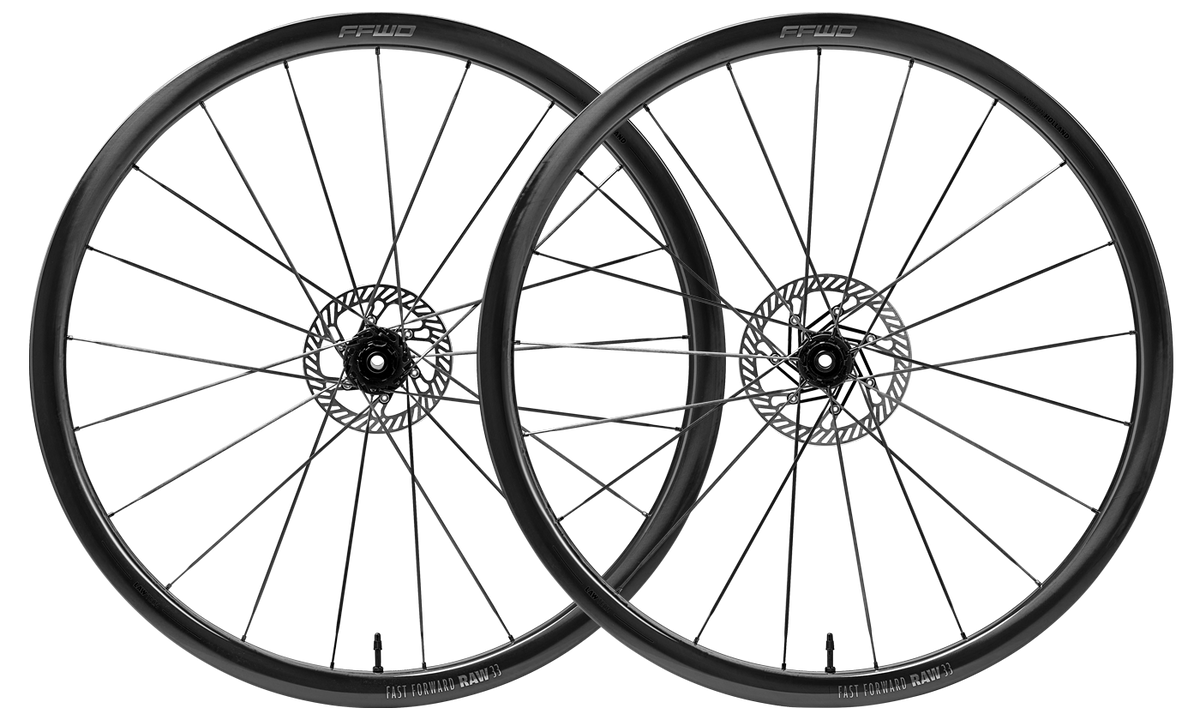The image shows two identical black bicycle tires against a plain white background, overlapping with the right tire positioned in front of the left. Each tire features a black center hub with a hole, surrounded by crisscrossing spokes that extend to the outer rim. There are 21 spokes on each tire, meticulously aligned towards the edges. Prominent on the rims is the branding "Fast Forward Raw 11" at the bottom and "FFWD" towards the top. Each tire has an air valve stem sticking out, prominently positioned. The overlapping arrangement creates an almost oval-shaped negative space in the middle of the image, emphasizing the structured symmetry and design details of the wheels.